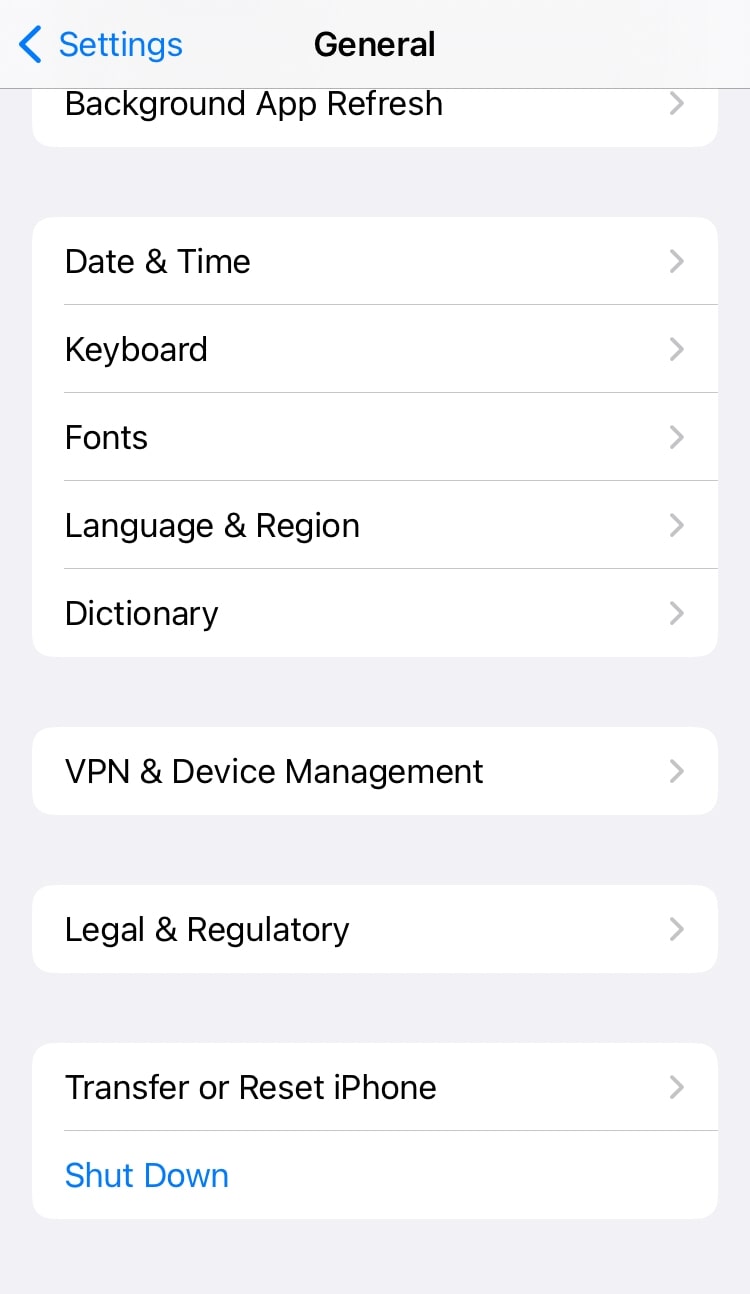The image displays a settings menu, likely from an iPhone, characterized by a clean, minimalist design. At the top left corner, there's a blue back arrow. The top of the menu features the word "Settings" in blue text, prominently displayed, with the subheading "General" in black text immediately beneath it. 

The list of options includes:
1. **Background App Refresh:** Cut off slightly due to scrolling.
2. **Date & Time**
3. **Keyboard**
4. **Font**
5. **Language & Region**
6. **Dictionary**

Each of these items is separated by single-pixel divider lines. After a small gap, another standalone option appears:
7. **VPN & Device Management**

Following another gap:
8. **Legal & Regulatory**
9. **Transfer or Reset iPhone**

At the bottom, another horizontal line separates these options from a blue-text link labeled "Shut Down."

The background color of the tabs is predominantly white, contrasting with the faint peach or pink hue of the entire menu background. This subtle coloring along with the structured layout creates a user-friendly interface, although the exact application or iPhone model isn't specified.